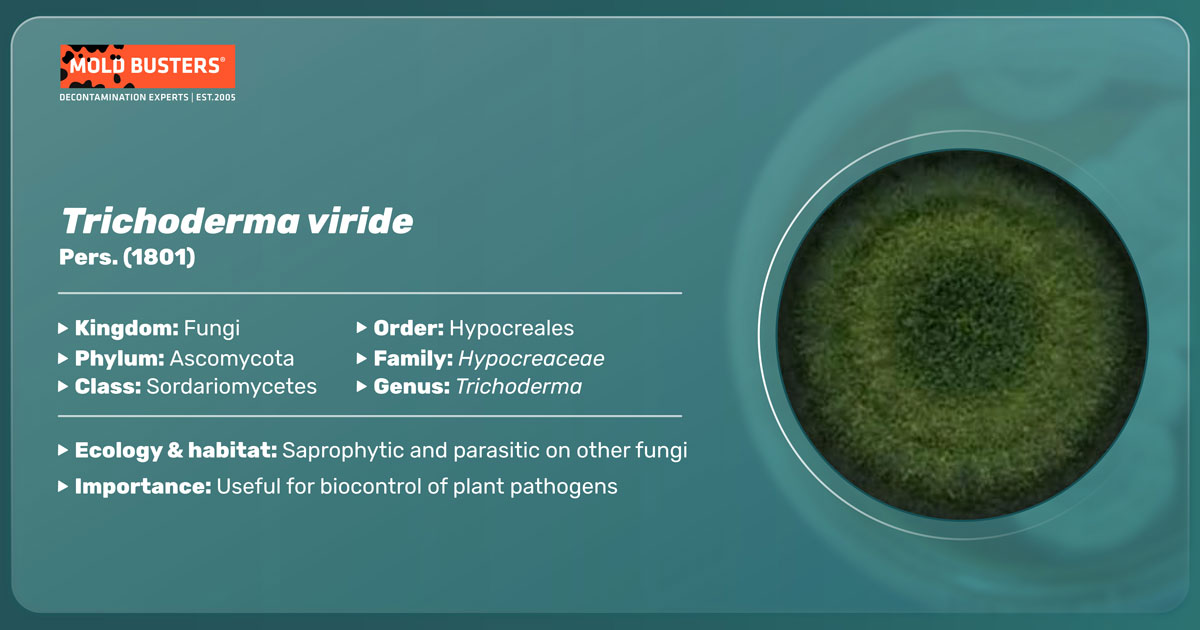The image is a fact sheet with a greenish-bluish background. Positioned in the upper left-hand corner is a rectangular section bordered in black and red, containing the text "Mold Busters" in white. Beneath this, the name of the mold is displayed: "Trichoderma viride." Below the mold's name, the designation "Per. (1801)" is listed. Further information is provided regarding the mold's taxonomic details, such as its kingdom (Fungi), phylum (Ascomycota), as well as its class, order, family, genus, etymology, and habitat. Additionally, the importance of the mold is discussed. Toward the center of the image, there is a green circle outlined in black, likely depicting the mold Trichoderma viride.